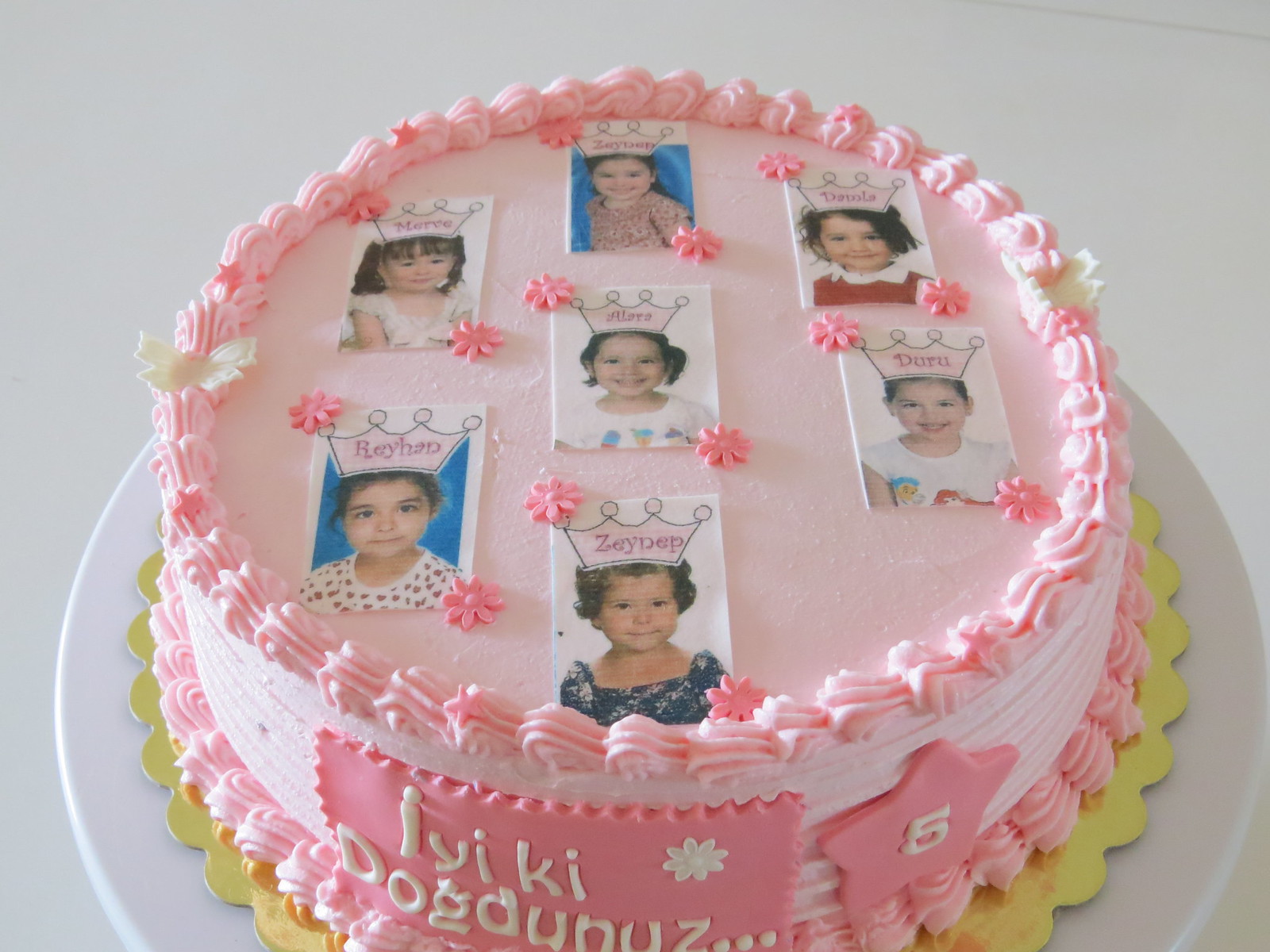The image is an indoor color photograph, showcasing a single-layer, pink frosted birthday cake from a slightly diagonal front angle. The cake is adorned with intricate pink piping along both the top and the base, which rests on a gold board with cloud-like undulations, all placed on a white ceramic plate against a white background. The cake prominently features a collage of edible photographs of seven young girls, each adorned with cartoon-like, pink crowns embellished with circular swirls ending in jewel shapes, each bearing the child's name. The front of the cake displays foreign text piped in white icing, with "IYIKI" on the top line and "DOGDYNUNZ" partially visible below, suggesting it might convey "Happy Birthday" in another language. There's also a pink fondant star with a white piped number five, indicating that this cake is for a shared birthday celebration for the girls, who are all likely turning five years old. The photographs are arranged in three columns—two on the left, three in the center, and two on the right—enhancing the cake's personalized and festive nature.